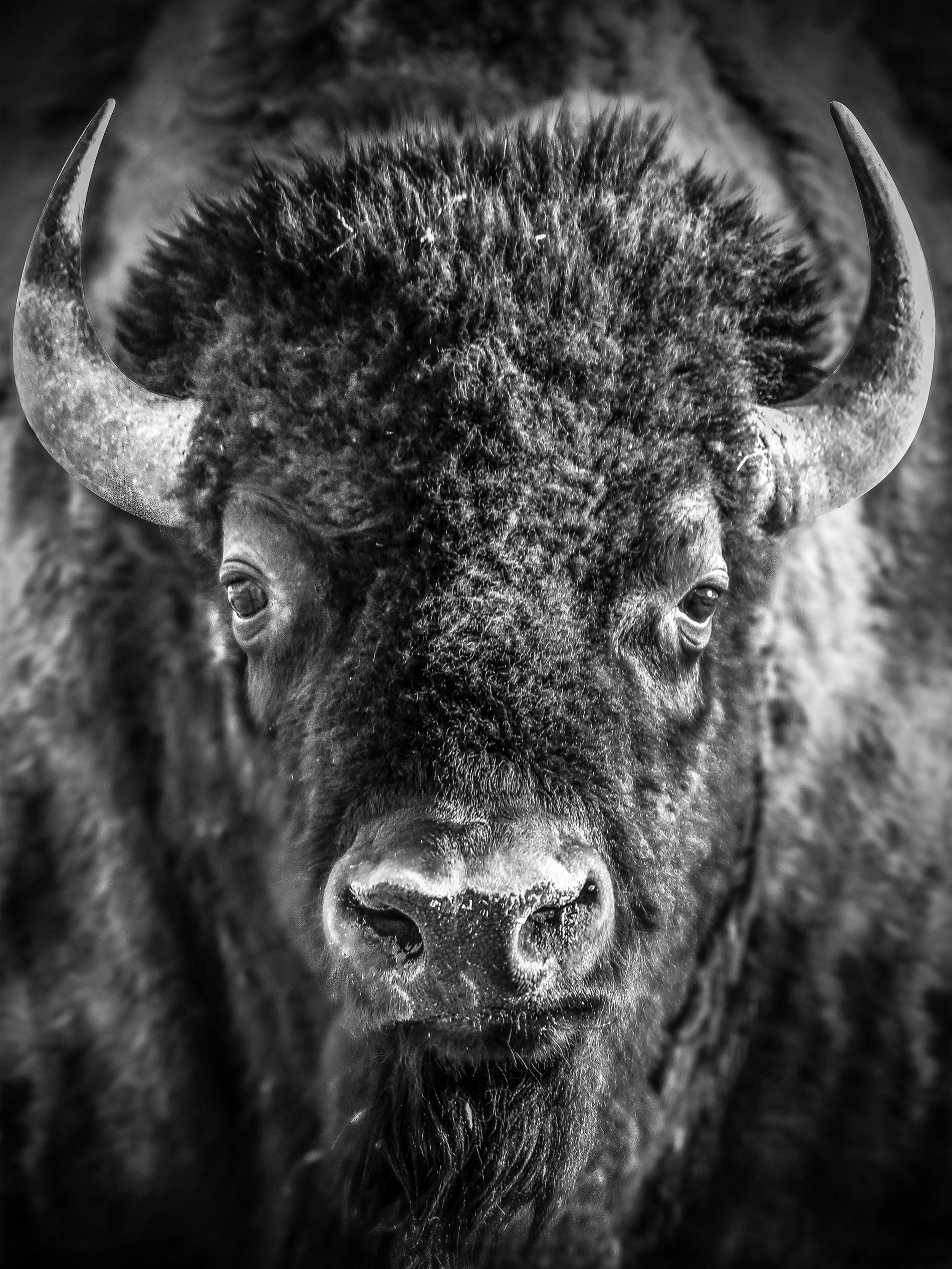This black and white photograph is a striking, close-up portrait of a bison. The image focuses primarily on the bison's head, which takes center stage with remarkable clarity and detail. The thick, textured fur covering its face and head is vividly captured, revealing the intricate patterns and contrasts of the fur. The bison's expressive eyes look directly forward, framed by powerful, upward-curving horns that start just behind the ears and narrow to sharp points. Below the large snout and mouth, a goatee-like tuft of hair hangs down, adding to the majestic presence of the animal. The background of the photograph is dark and blurred, creating a dramatic contrast that highlights the bison's formidable features and the artistry of the photography.